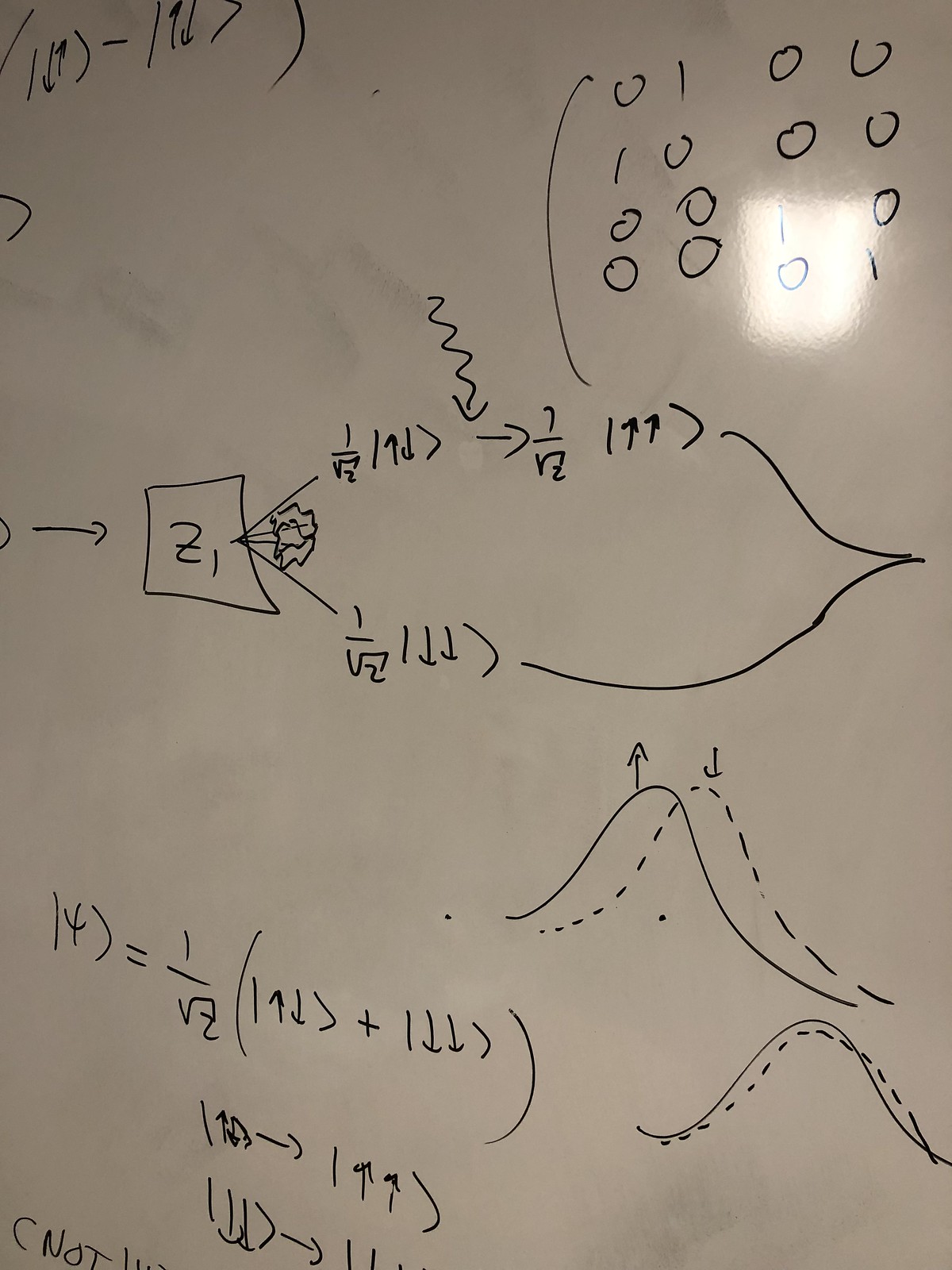In this detailed whiteboard illustration filled with mathematical expressions, the wear and marks of previous erasures are evident, adding to its character. At the top right, a neatly drawn 4x4 grid entirely composed of zeros and ones is visually striking. The arrangement seems methodical: 0 1 0 0, 1 0 0 0, 0 0 1 0, and 0 0 0 1, bearing a resemblance to a Sudoku puzzle or perhaps a matrix.

Beneath this grid, an arrow directs attention to a box labeled "Z1," which branches out into complex formulas, one situated above the other. These formulas extend into two lines that converge at a single point.

Moving downward, two parabolas dominate the scene - the solid one accompanied by an arrow pointing upward, and a dotted one with an arrow directed downward. Below, a similar illustration is repeated, with the solid and dotted lines closely overlapping.

In the bottom left corner, the notation "14" followed by a parenthesis catches the eye. This is trailed by an equals sign and an expression resembling "1 over the square root of Z," enclosed in parentheses with an intervening formula. Two additional formulas are discernible beneath this notation. Just at the periphery, partially obscured, the word "NOT" in parentheses hints at more mathematical considerations cut off from view.